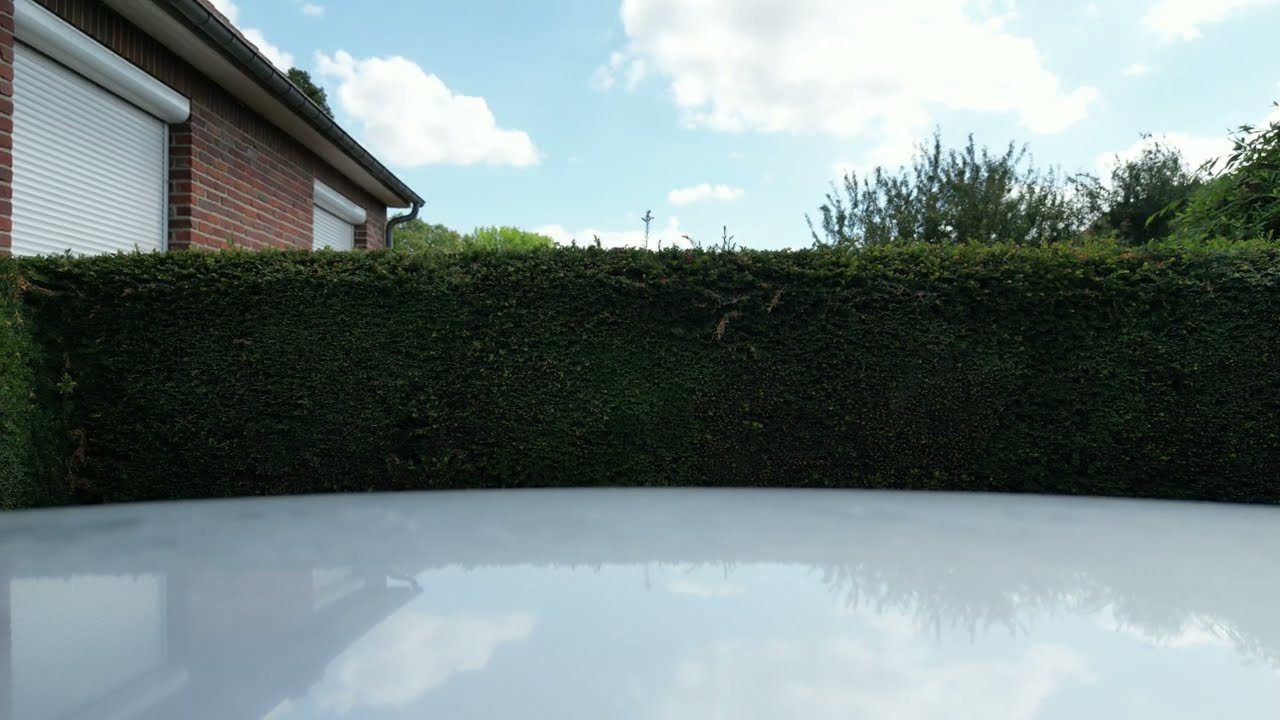The image depicts a highly reflective, milky surface likely belonging to a white or silver car. This surface mirrors the blue sky with scattered light clouds and sunlight filtering through from the upper right corner. Behind the car, a dense, luscious green hedge spans the entire horizontal axis of the photo, providing a well-maintained barrier. On the left side of the image, behind this hedge, stands a red brick house that appears to feature white outdoor roll-up metal shades over its windows, which could be either for hurricane protection or resemble small garage doors. In the background, beyond these elements, there's a mix of lighter and darker green trees, with a thin power pole rising into the skyline, blending into the partially cloudy, mostly blue sky.